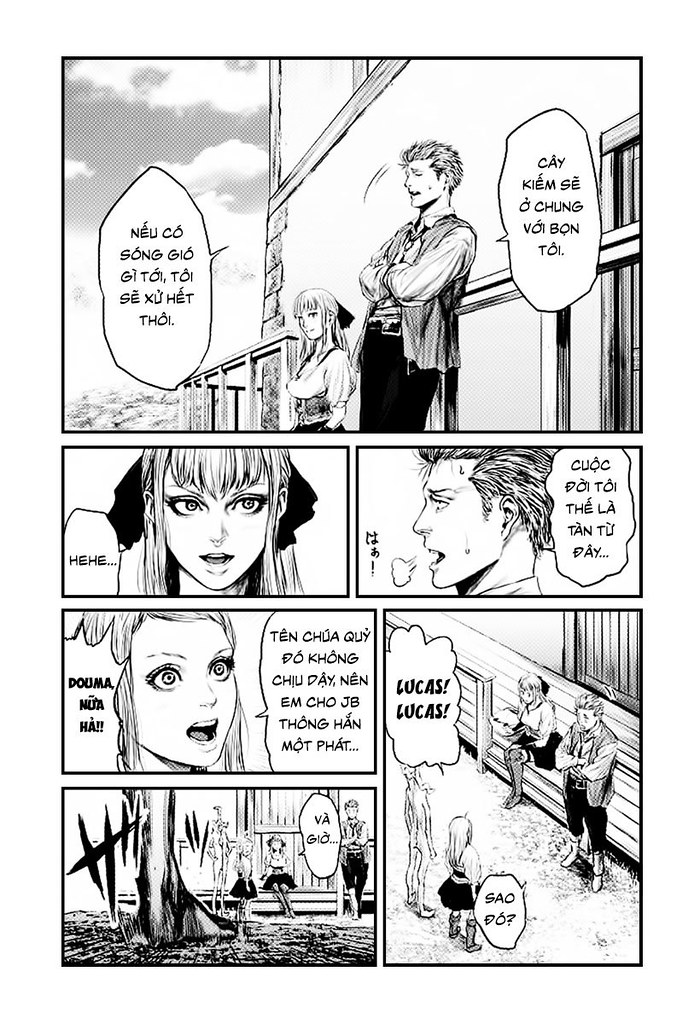This black and white comic strip, possibly inspired by Asian animation, consists of six panels. In the top rectangular panel, a man and woman are seen outside, leaning against a fence in front of a building. The man, with his arms crossed, is talking to the woman who stands with her hands at her sides, long hair and bangs cascading down. Their conversation is in a language that appears to be Vietnamese.

The next row features two panels: to the left, a close-up of the woman as she says "hee hee," her long hair prominently displayed; to the right, a close-up of the man with a puff of smoke or breath coming out of his mouth, his face turned to the side, accompanied by more Vietnamese text.

Beneath these, the next row shows the woman again, her eyes wide and mouth open in surprise, with another caption in Vietnamese. Adjacent to this, the man is seen again, standing against the fence, while the woman has taken a seated position next to him. A young girl and another character are in front of them, possibly engaged in conversation with the initial pair.

The bottom row features a group of children sitting next to a tree, marked by a distinctive slash with four lines. In this scene, the children call out "Lucas, Lucas," seemingly addressing the man, who is implied to be named Lucas. The ongoing dialogue remains in Vietnamese, adding an element of mystery to their interaction.